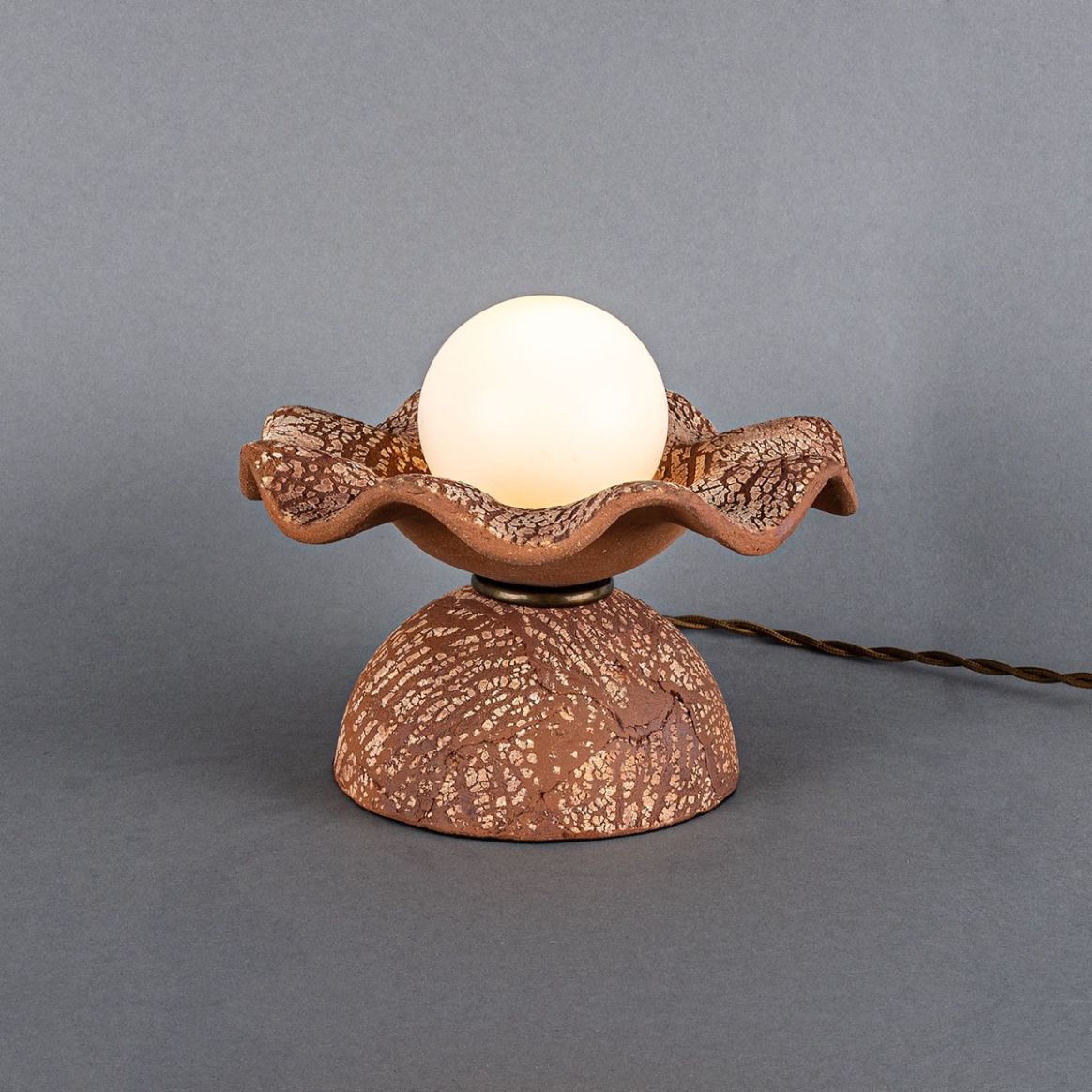This image features a distinctive lamp, centrally positioned, exuding a warm glow from its smooth, round, white orb bulb. The lamp is set against a gray background, resting on a gray surface. The lamp stands out due to its unique base, which resembles a blooming flower or an oyster shell cradling a pearl. The base is crafted from a rustic, clay-like material with intricate beige textures and a crackled finish, giving it an antique, pottery appearance. The frilly, wavy edges of the base add to its floral or shelly aesthetic. The lamp's twisted brown electrical cord extends from the setup towards the right side of the image, adding a textured contrast to the sleek orb. The merging point between the frilly top and the smooth, rounded base is marked by a subtle gold plate, lending a touch of elegance to the overall design.